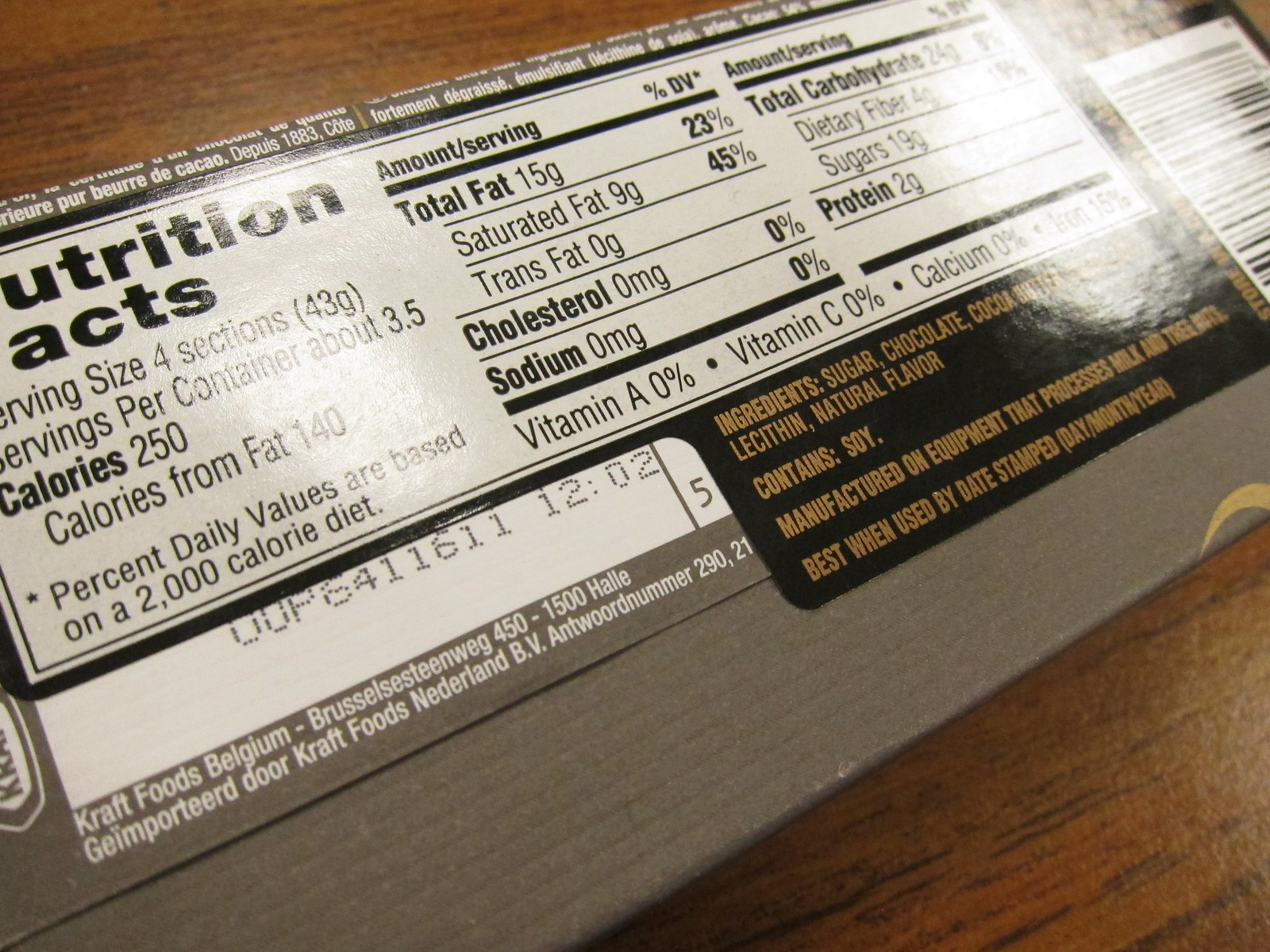This close-up image captures the back of a chocolate bar, wrapped in brownish paper. The partial view of the label shows "Nutrition Facts," though the "N" and "F" are partially cut off. The ingredients are printed in orangish lettering and list: sugar, chocolate, cocoa butter, lecithin, natural flavor, with a note that it contains soy and is manufactured on equipment that processes milk and tree nuts. There's a reminder that the product is best when used by the date stamped in the format (day/month/year).

Detailing the nutritional information, the label states that each serving size is four sections, approximately 43 grams, with about 3.5 servings per container. Each serving contains 250 calories, with 140 calories from fat. A note clarifies that the percent daily values are based on a 2,000 calorie diet.

In the bottom left corner, the label features white lettering identifying the manufacturer as Kraft Foods, located at Brussels Steenweg 450, 1500 Halley, Belgium. Additional text, possibly in German or another language, mentions that the product is imported by Kraft Foods Nederland BV, indicated by the import code "Antwoord Number 290." This detail suggests the chocolate bar was produced in a European country.